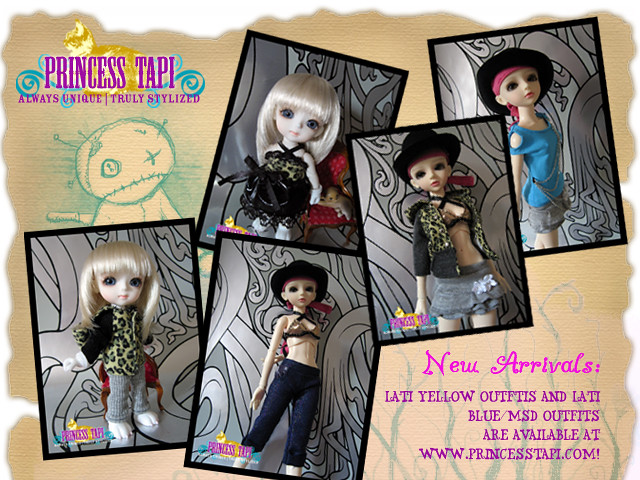The image showcases five unique Princess Tappy dolls, strikingly reminiscent of Bratz dolls, with a promotional overlay. Positioned in five distinct panels against a black textured background, these dolls sports various fashionable outfits, ranging from casual to more formal styles. Two dolls have platinum blonde hair, one wearing a dress, and the other a suit and pants, while the remaining three, with pink hair and wearing hats, are dressed in casual attire including jeans, jean shorts, skirts, and jackets. The top left corner features the text "Princess Tappy, Always Unique, Truly Stylized" in pink, set against a backdrop of a voodoo-like doll with pins and stitches, adding an eerie element. The text "New arrivals, Ladi Yellow outfits and Ladi Blue MSD outfits are available at www.princesstappy.com," appears at the bottom right in purple. The dolls' faces, marked by dark eyes and slightly unsettling expressions, hint at their collectible nature, possibly intended for a more mature audience.